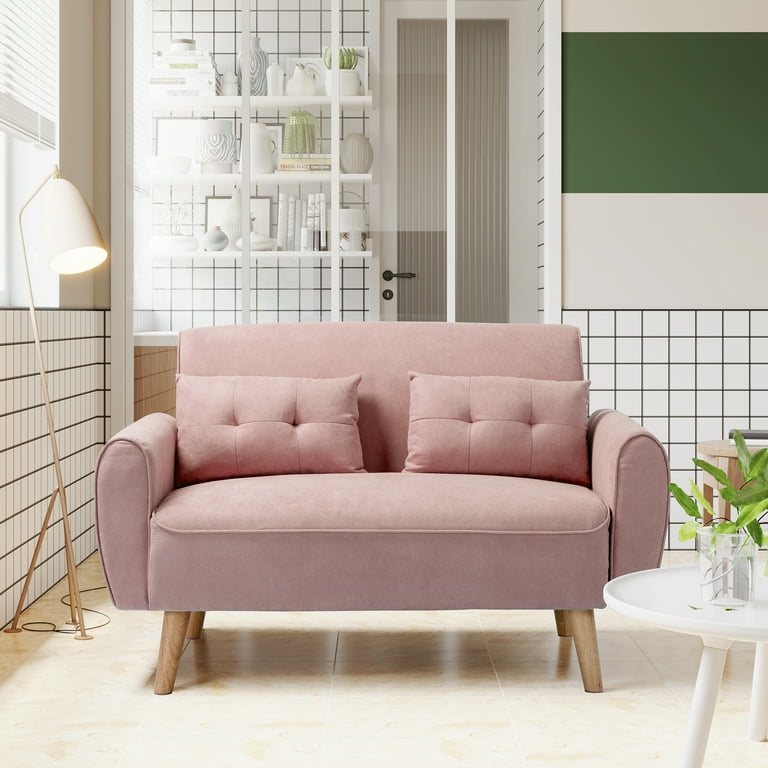The image captures a staged room designed to highlight a light pink two-seater couch, probably intended for a commercial online platform such as a catalog or website. The couch, with tall armrests on either side and cylindrical wooden legs positioned on a yellow and brown tiled floor, is adorned with two square pleated pillows. Adjacent to the couch, on the left, is a low lamp, and on the right stands a small side stool holding a green-leafed potted plant. The room's walls combine white tiling at the bottom with a white or gray paint above. In the background, a glass wall reveals a shelf system filled with decorative items, including flower vases, books, small picture frames, and ceramic cups. The predominant colors are cream, brown, shades of pink, green, and white, lending the scene a cozy and aesthetically pleasing ambiance.